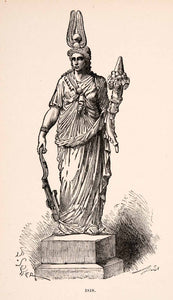This detailed line drawing depicts a statue of a deity adorned with intricate details. The figure, likely a woman, is garbed in ornate robes, reminiscent of traditional attire with possible cultural influences. She dons a crown, described as having two horns merging at the top with a ball in the center. The statue holds a crossbow in one hand, while the other hand grasps a decorative object, possibly a scepter or a stalk of flowers. Multiple necklaces and bracelets embellish her figure, adding to the rich ornamentation. The grayscale drawing accentuates shadows, contributing to the depth and texture of the artwork. A partially illegible signature hints at the artist's identity.